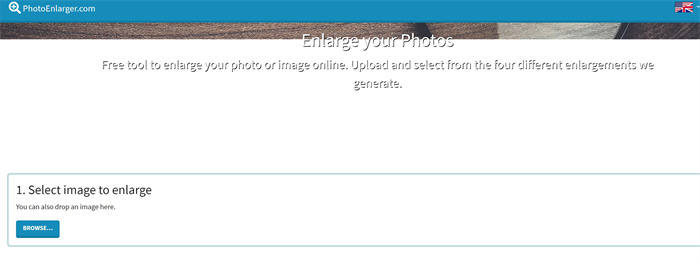This image is a screenshot of a computer screen displaying a web page for a photo enlargement tool. At the top of the screen, there's a prominent navigation bar labeled "Photo Enlarger," accompanied by an icon designed for enlarging photos. Just below this bar, there's a wood-textured strip with a semi-transparent overlay that reads "Enlarge Your Photos." Further below, there's a clear description of the service: "Free tool to enlarge your photo or image online. Upload and select from the four different enlargements we generate."

In the center of the screen, a white rectangle serves as the upload area, marked with a blue button containing white text that says "Upload Your Document." This button doubles as a drag-and-drop zone for images. The upload section is clean and uncluttered, offering a single, straightforward interface for user interaction. Additionally, in the top right corner, a British flag icon suggests language or regional settings for the website.